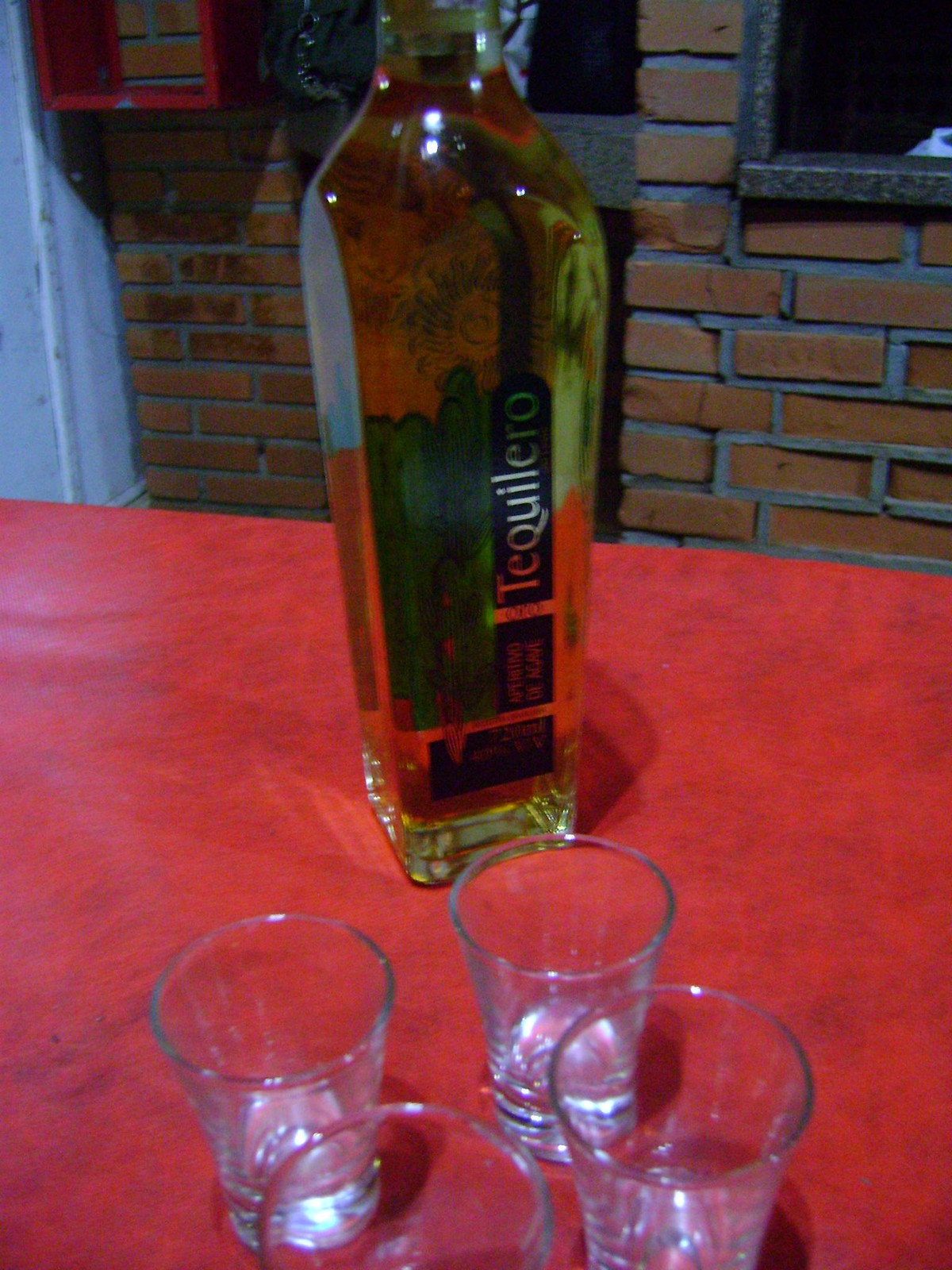This is a vertical rectangular color photograph taken indoors, possibly under harsh fluorescent lighting. The image centers on a red tablecloth-covered table where a tall, slender bottle of tequila, labeled "Tequilero" in white vertical lettering on a black bar, is positioned. The top of the bottle extends slightly above the middle of the photograph. In front of the bottle, clustered together, are four clear shot glasses, presumably empty, with the bottom-most glass partially cut off by the edge of the image. The background features a brown brick wall with gray mortar, and a red box resembling a fire extinguisher case is mounted on the upper left side. Additionally, there appears to be a stone or concrete shelf and possibly some service windows within the brick wall.